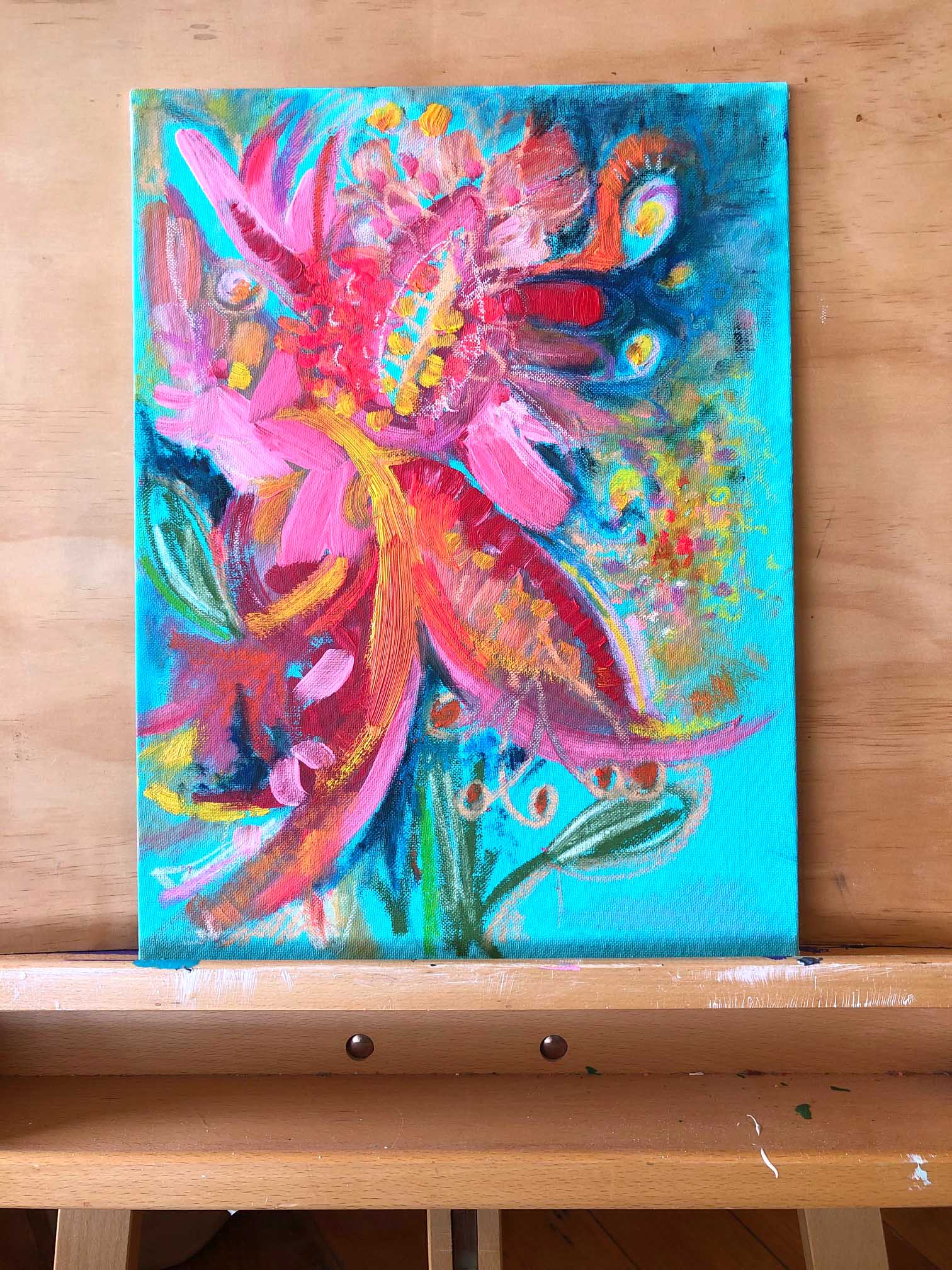In this image, we see a detailed and colorful painting of flowers positioned at the center on a wooden easel with a lighter color. The background of the canvas features a light blue hue with darker blue swirls visible in the top right corner. Prominently displayed in the painting is a large flower with pink petals surrounding a yellow center. The flower is connected to a green stem adorned with a substantial green leaf on the right side. The easel, which has a shelf portion at the bottom, stands on three visible legs, with the floor beneath it also included in the frame. The painting overall exudes a vibrant palette consisting of various shades of orange, yellow, red, blue-green, blue, green, and darker pink.